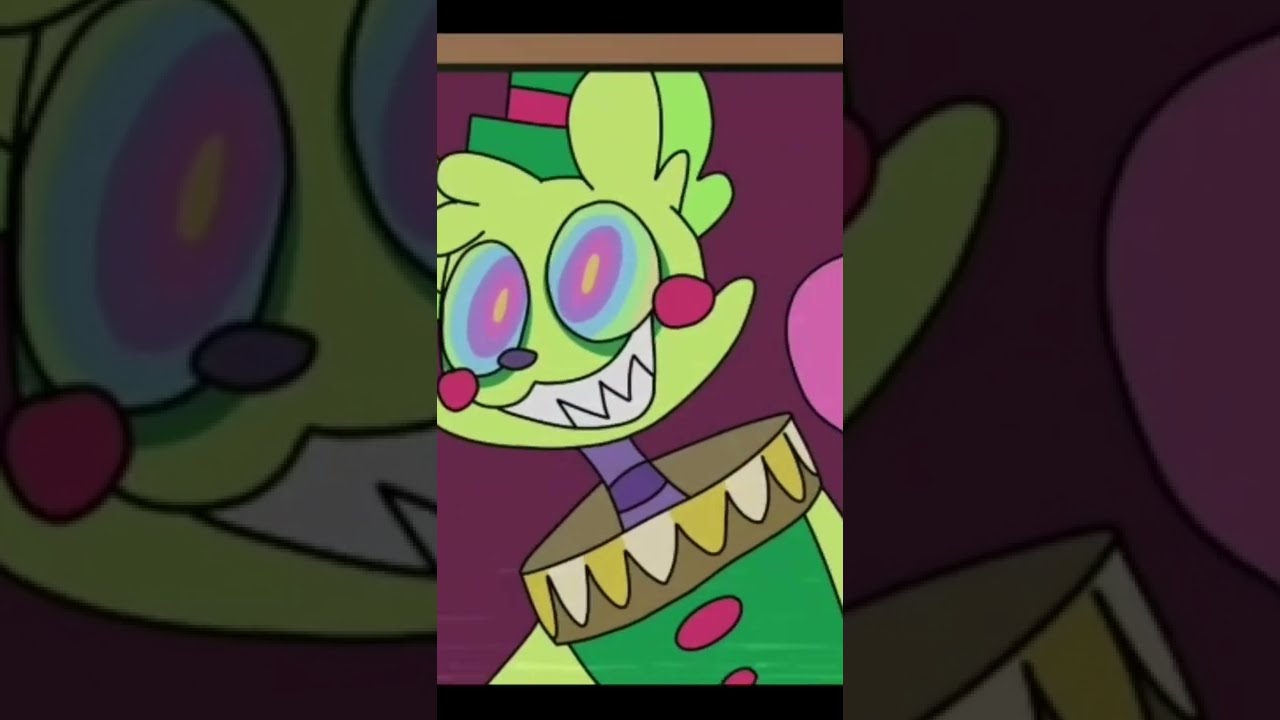The image depicts a vibrant piece of digital artwork, possibly animated and resembling a scene from a children's cartoon or movie. The central character, placed prominently in the middle of the composition, exhibits a whimsical design. This character has a green cylindrical body adorned with pink circles and wears a green and pink hat. The face is quite expressive, featuring large, multi-colored eyes (yellow centers, red rings, black outlines, and blue edges), with a wide smile that shows teeth shaped like a jagged 'W'. Purple circles accentuate the cheeks, adding to the character's playful appearance.

Around the neck, the character wears what appears to be a purple ruffle, contributing to the colorful attire, which includes a green shirt decorated with a large pink button at the top and a smaller pink button below. Light yellow arms extend from the body, adding to the cartoonish look.

The background complements and emphasizes the main figure, presenting an enlarged, darker portion of the same image, ensuring the details on the right side of the character's face and the light purple half circle on the purple backdrop are more pronounced. This dual-layered presentation creates depth and enhances the visual impact of the artwork, drawing attention to the character's quirky and vivid features.